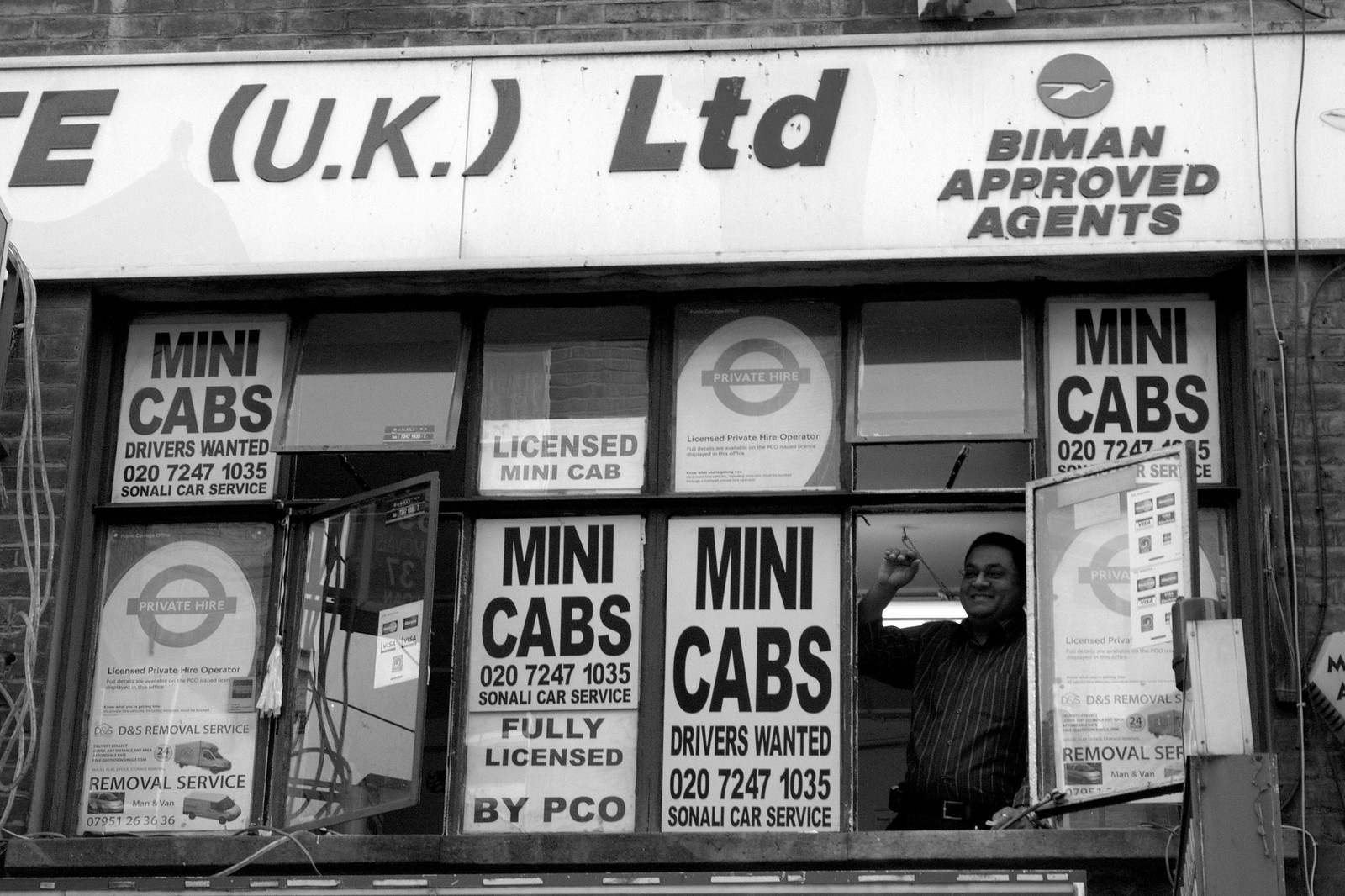This black and white photograph captures a storefront in the UK, marked by a sign overhead that reads "UK LTD" and "Byman Approved Agents." The storefront features multiple smaller signs and posters in the windows, which consistently advertise for mini cab drivers with text reading "Minicabs Drivers Wanted," "Fully licensed by PCO," and the contact number "020-7247-1035" for Sonali Car Service. A man is seen standing in one of these open windows, with his right arm raised and smiling, adding a welcoming, perhaps pointing gesture toward the signage. The repetition of the minicab service posters and the setup of the window evoke an old-fashioned, approachable service point, similar to a drive-up window at a fast-food place.